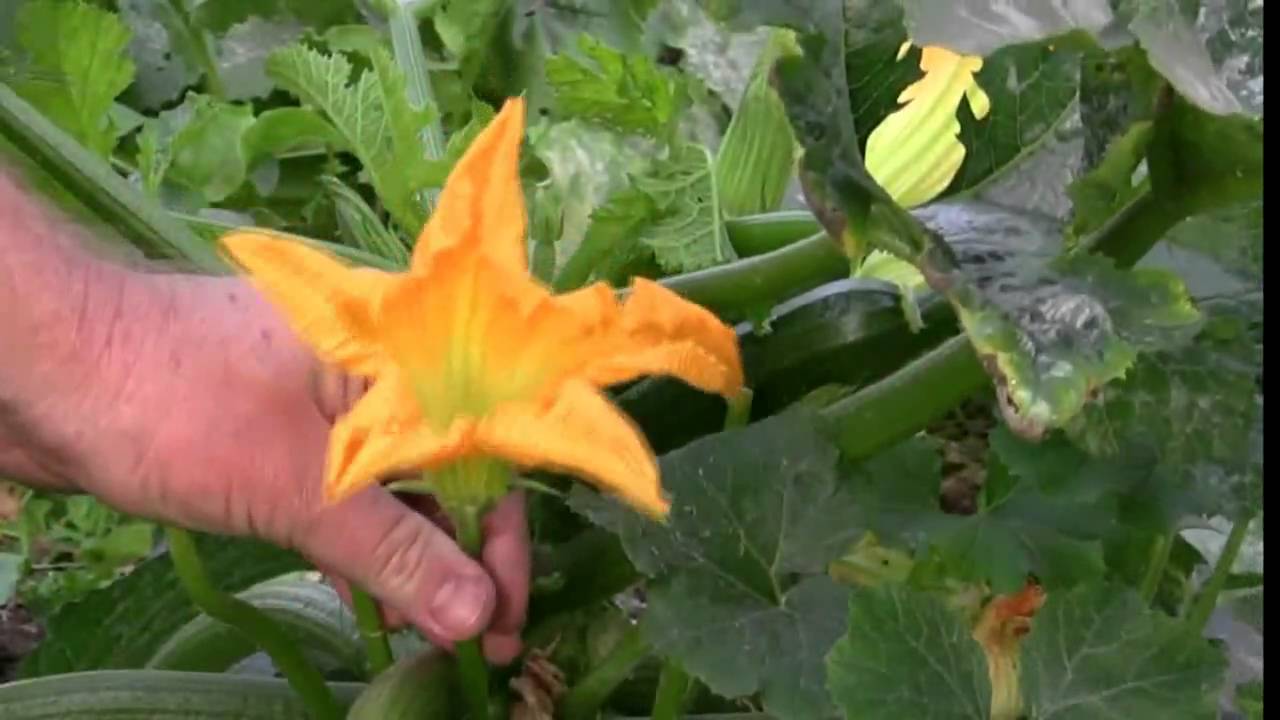The image captures a senior adult's hand coming in from the left side, in the act of picking an orange star-shaped flower that appears to be somewhat dry. The hand is grasping the thick stem of the flower, positioning itself to pluck it. The flower, with its inwardly curled, bright orange petals, stands out among the lush, dark green leaves surrounding it. These leaves resemble those of salad greens, with some being long and jagged while others are smooth. In the background, additional greenery can be seen, along with a few green pots and a subtle gray surface, contributing to a slightly blurred effect, likely due to the motion of the hand in the image. Overall, this detailed scene highlights the contrast between the vibrant flower and the rich green foliage that encircles it.